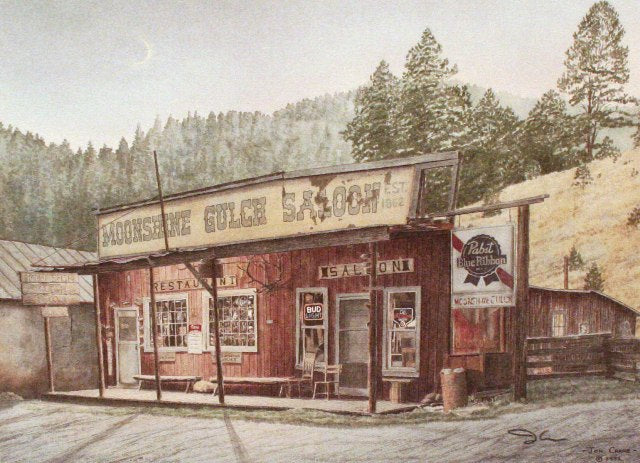This detailed illustration captures an Old West countryside scene, focusing on a run-down, one-story wooden building labeled "Moonshine Gulch Saloon." The building, painted red with a white door, has two front windows labeled "Restaurant" and a separate door on the right marked "Saloon." Above the building hangs a light brown, weather-beaten sign that reads "Moonshine Gulch Saloon." Additionally, there's a Pabst Blue Ribbon advertisement near the saloon door. The setting appears transitional between day and night, with a subtle gradient from dark to light in the sky. A crescent moon is visible, adding to the vintage ambiance. In the background, a hill covered with dense pine forest creates a natural, rugged backdrop. The building features a porch with an awning supported by wooden poles, enhancing its rustic charm. This color sketch or painting effectively portrays a nostalgic, Western-style roadside bar, evocative of a bygone era.